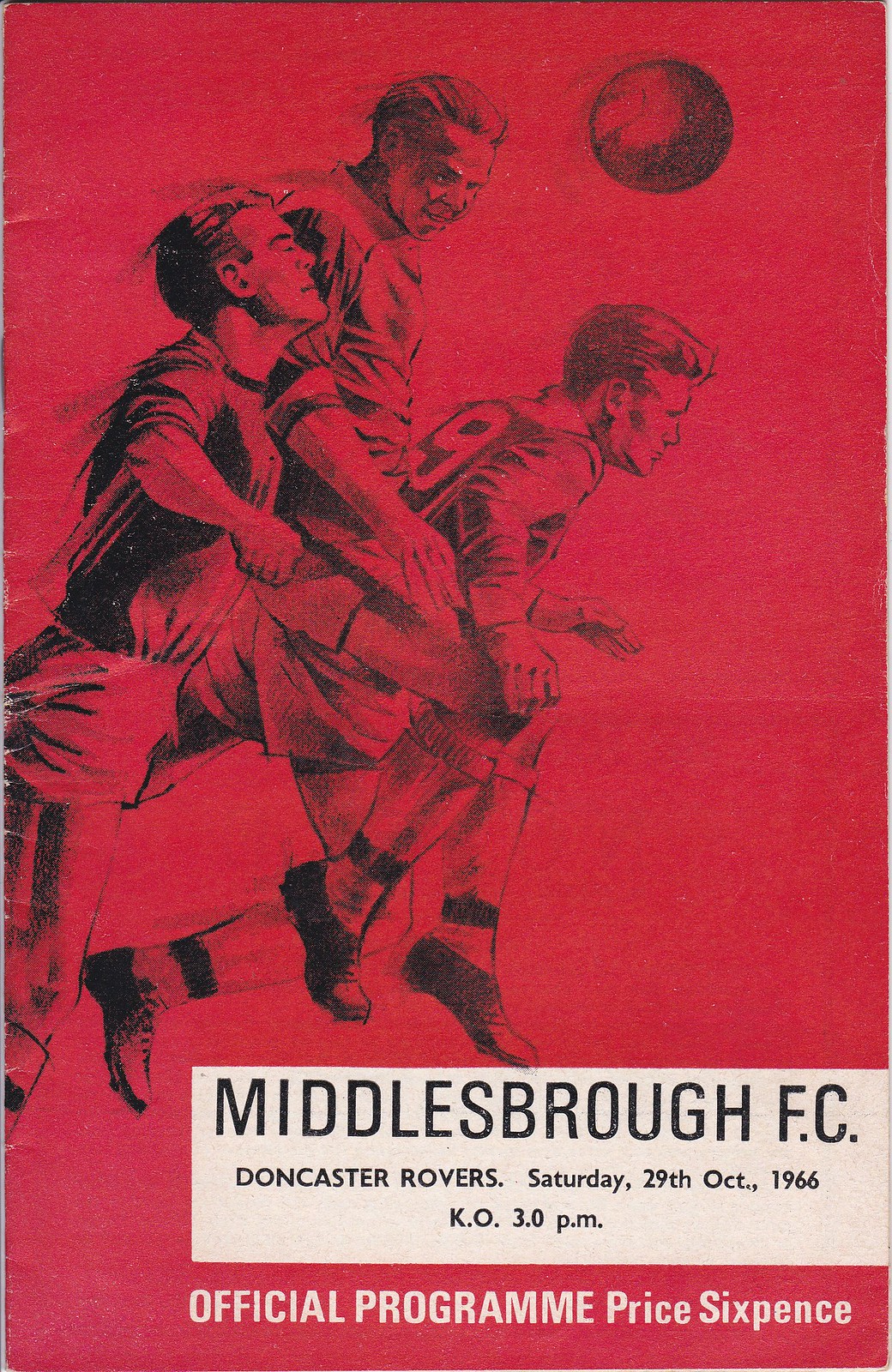The cover of the magazine displays an illustration of three soccer players seemingly in midair, likely jostling for position to head a ball into the net. The soccer ball is positioned near the top right corner of the image. The composition centrally focuses on the players, all depicted in red hues which match the red background, lending a unified and striking aesthetic to the cover. The entire image, including the players' jerseys and faces, is tinted red, giving it a monochromatic and intense appearance. Some creases and wrinkles are evident on the left side and down the middle of the page, suggesting age and wear of the magazine. At the bottom of the cover, a cream-colored rectangle features bold black text reading “Middlesbrough FC” followed by “Doncaster Rovers,” “Saturday 29th October 1966,” and “KO 3.0 PM.” Below that, in white text against the red background, it reads “Official Program Price 6 pence.” This detailed, nostalgic cover captures a historical soccer match program dated 1966.